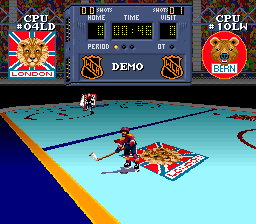Screenshot of a vintage video game featuring a pixelated ice hockey match in a brightly lit arena. The predominantly blue ice rink is central to the scene. At the top of the screen, team names "London" and "Bern" (with "B-E-R-N" clarified) are displayed, indicating a face-off between the London Lions and Bern. The scoreboard shows a 0-0 tie, reflecting it in another language as "W-L-H" alongside a hockey shield icon. The left side of the screen is adorned with blue and yellow arena decorations. A time stamp reads "00:45," suggesting the first period is nearly half over. Notably, the Bern team has registered one shot on goal, although the score remains even at 0-0.